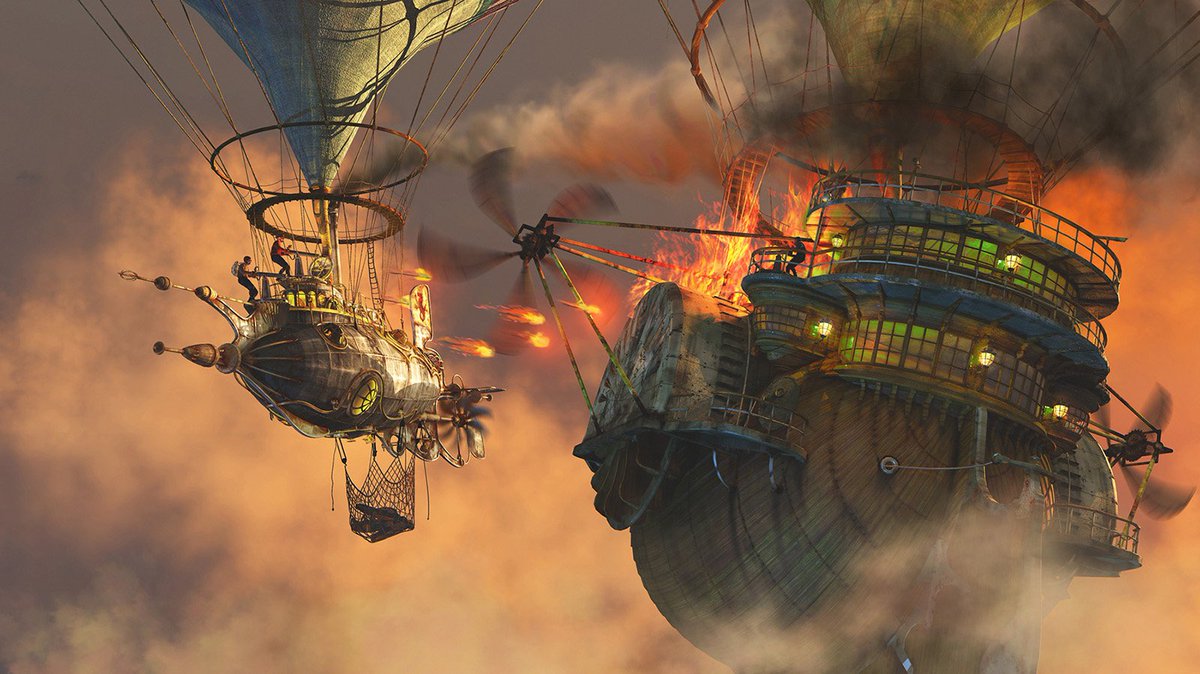This image is a finely drawn, steampunk-style depiction of a dramatic aerial battle between two airships, reminiscent of a scene from a graphic novel, television show, or video game. The larger airship, positioned on the right, is reminiscent of a colossal pirate ship suspended by a massive hot air balloon. It has two decks lined with bars on the windows and is equipped with cannons and propellers on its sides. The ship is glowing green from within, possibly from the captain's quarters at the front. The deck is engulfed in red and orange flames with dark smoke pluming skyward, indicating it has sustained heavy damage from the assault. Two shadowy figures are present on the deck, one of whom is attempting to fire back.

On the left, a smaller airship, also held aloft by a balloon, is actively engaging the larger vessel. This smaller craft, metallic and possibly with a slight watermelon shape, features rotor blades and a prominent net hanging beneath carrying some unknown cargo. At least two men can be seen manning weapons, firing fiery projectiles and flaming arrows at the larger airship, causing significant destruction.

The sky in the background is filled with clouds and smoke, enhancing the gritty, chaotic atmosphere of the mid-air clash. The fiery projectiles from the smaller ship light up the scene, casting an ominous glow over the entire battle. The overall color palette consists of deep reds, blacks, and oranges, which heighten the intensity and drama of the scene.